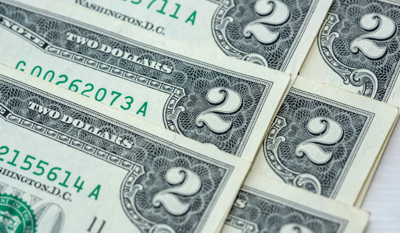The image showcases a pile of six overlapping $2 bills, with only the upper right corners of the bills visible. The arrangement of the bills shows the ones closer to the viewer on top, overlapping those further back. Each bill displays the number "2" prominently in the upper right corner, running diagonally down the right side of the image. The top bill partially reveals the series number "711-A" in green ink, while the second bill shows "G00262073A" in green, and the bottom bill, partially cut off, displays "2155614A" in green. Underneath this number in black text, "Washington, D.C." is visible, but the "WAS" is truncated. The texture suggests that each visible bill might be part of a small stack, adding thickness to the pile. The distinctive green serial numbers and the mention of "Washington, D.C." highlight the historical aspect of these rarely seen $2 bills.